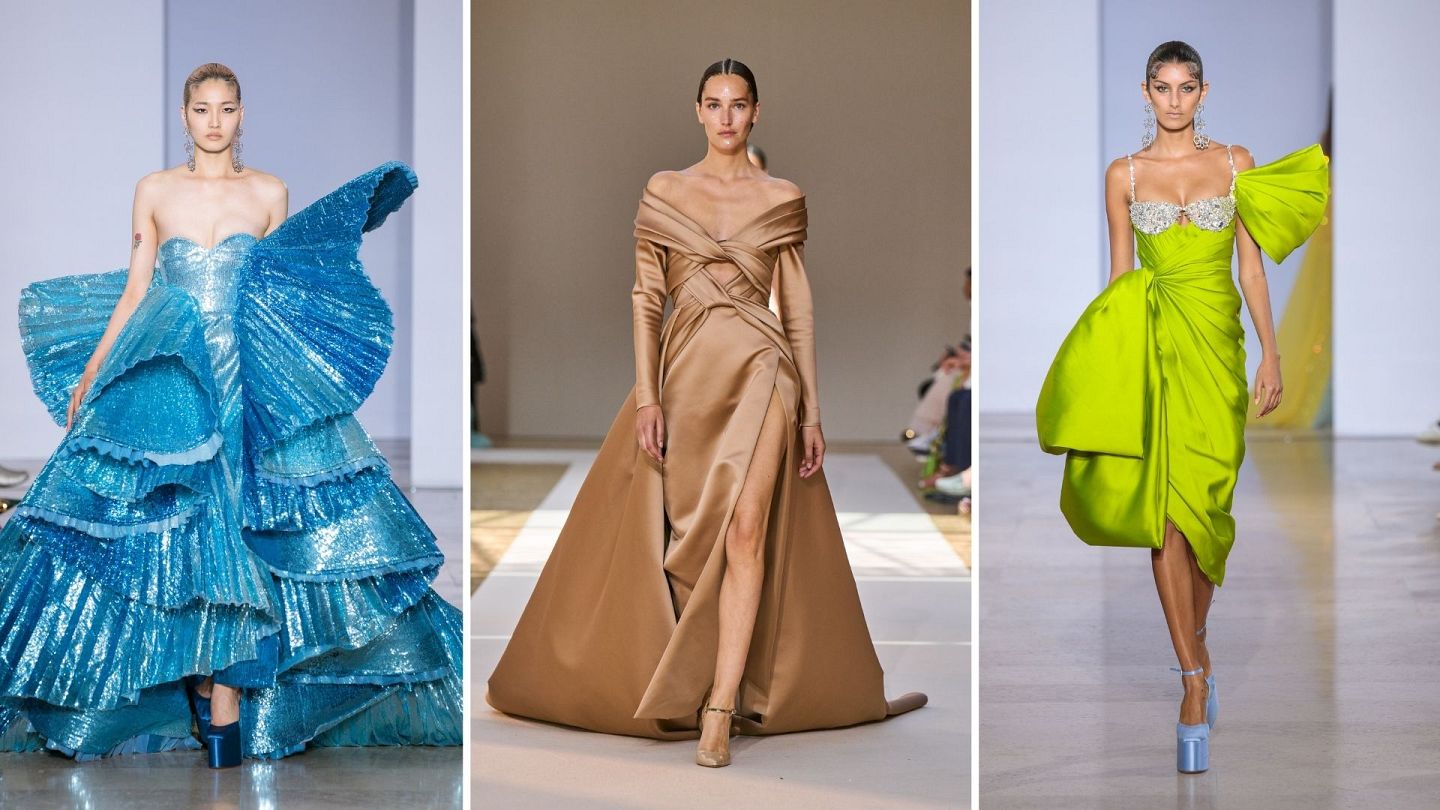The image captures a vibrant scene from a fashion show, showcasing three stunning models. The backdrop for the models on the left and right features blue tones with door-like shapes, while the center background is brown. Starting from the left, the first model wears an elaborate, textured blue dress reminiscent of something from *The Little Mermaid*. She pairs it with dark blue heels, her hair pulled back into a ponytail, revealing dangly earrings and a tattoo on her right arm. The center model is in a silky, brownish-gold dress with an open slit at the bottom, complemented by beige heels and slicked-back hair. On the far right, the model dazzles in a bright lime green dress with a glittery silver chest covering, paired with light blue heels. All the women have fair skin, perfectly styled hair, and are walking on a grayish-white floor, their makeup skillfully applied, emphasizing their striking features in this high-quality image.